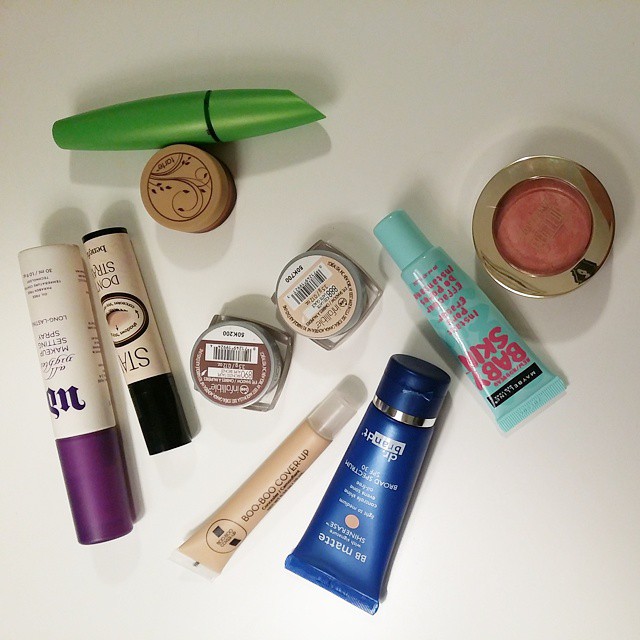A neatly arranged collection of beauty and skincare products is displayed on a pristine white countertop. The assortment includes a variety of makeup and skincare items, each meticulously placed. Central to the collection is a green tube, complementing a light blue tube with a matching light blue cap labeled "Baby Skin." Another notable item is a dark blue tube with a dark blue cap, though the label is not legible. Among the collection is also a light tan tube with a clear lid, clearly marked as "Boo-Boo Cover-Up." Surrounding these key items are several other beauty products whose labels are not visible. The items are predominantly designed for women and include makeup, skincare, and blemish cover-up products, indicative of a personal collection carefully laid out for easy access and use.